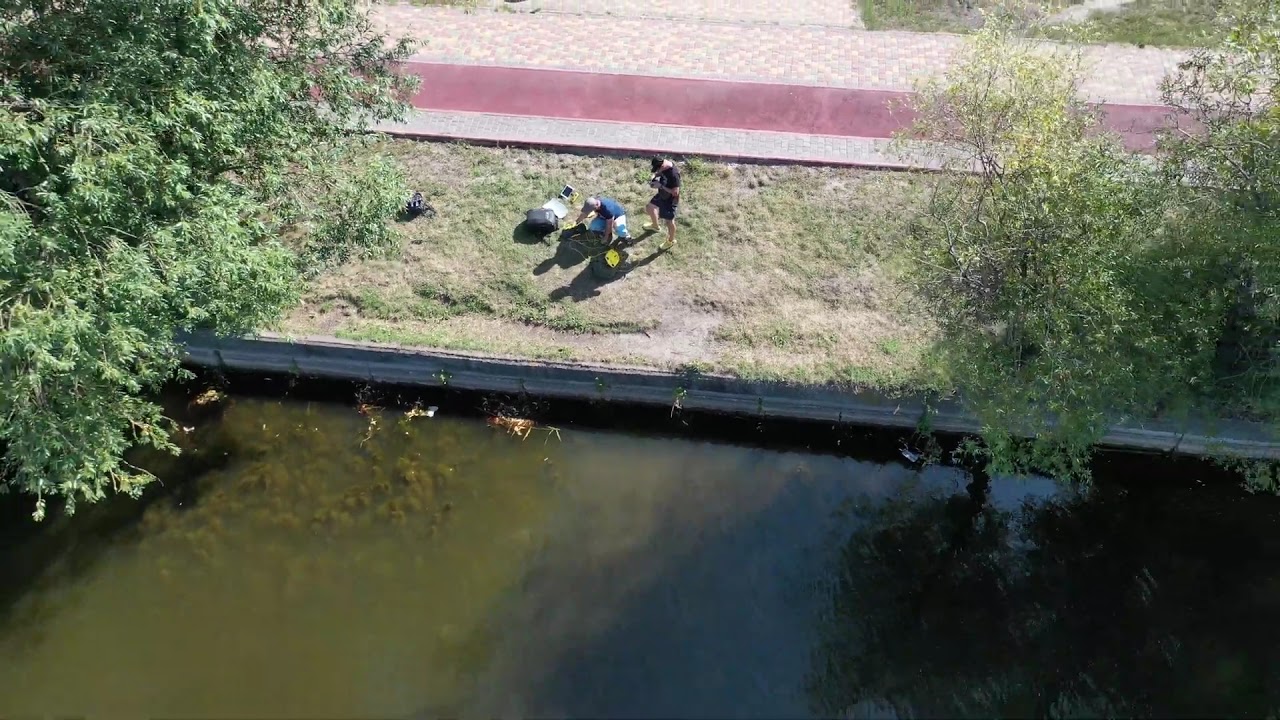In the center of the image, there are two men on the edge of a murky, green body of water, which takes up about 40% of the lower part of the picture. The man on the right is standing, wearing a dark shirt, dark shorts, a dark hat, and white shoes. His head is bent down and his hands are held in front of his chest as he examines something. The man next to him is down on his hands and knees, clad in a blue shirt, white pants, and a white hat, seemingly fiddling with a few objects on the ground. Their shadows stretch towards the bottom left of the image. Behind them is a bright amber walkway, constructed from various types of stones and flanked by rock-built formations. The left side of the image is dominated by a thick tree with dark green leaves, while the far right hosts a dense bush with yellow-tinged leaves. The overall scene appears to be captured from a high vantage point, possibly a drone.